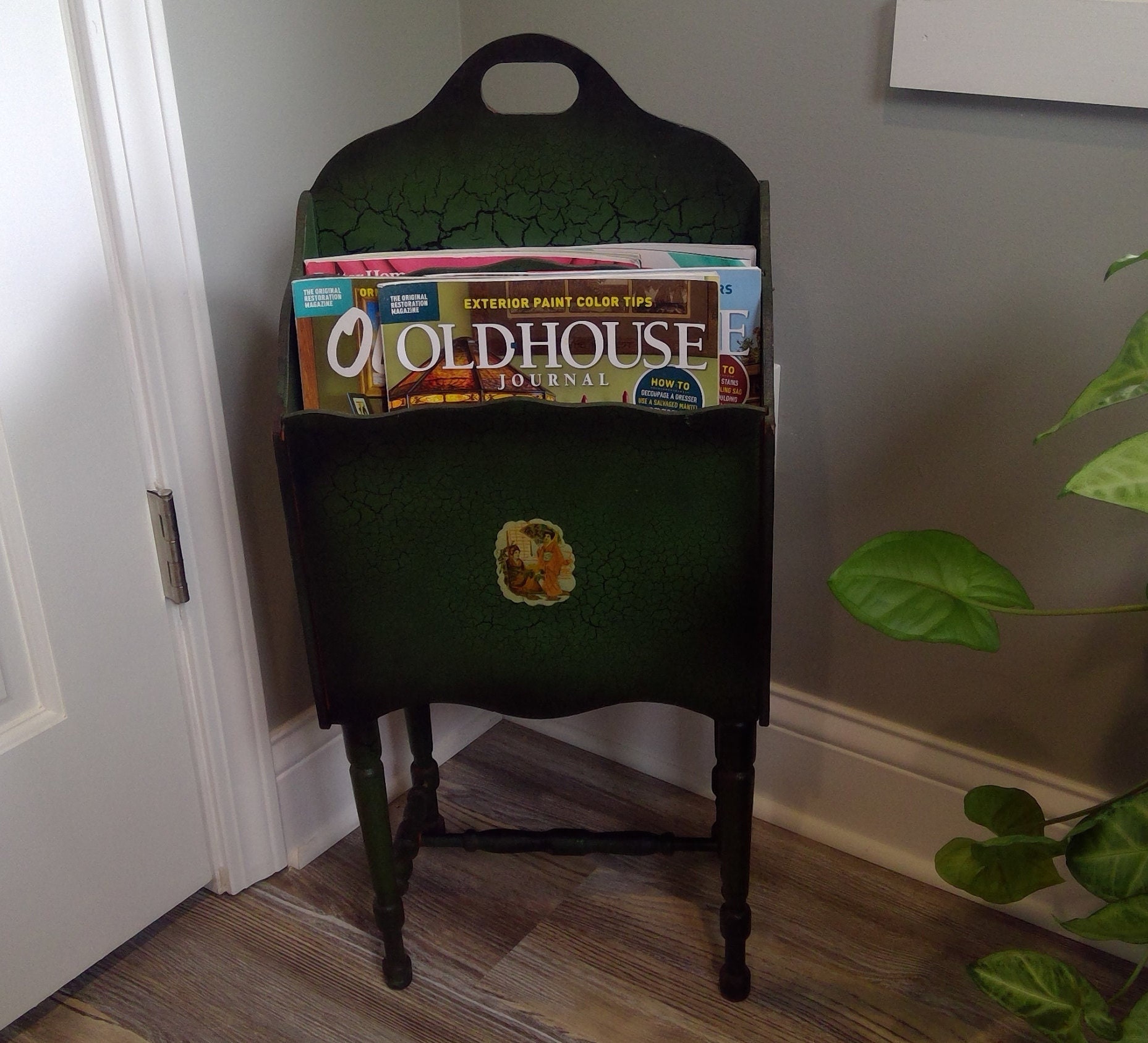In the corner of a room, a magazine stand made of wood and painted a dark, possibly black, color stands out. Positioned against a grayish-colored wall, the stand features a small image on its front panel, which appears to depict two women dressed in traditional kimonos with large fans. The wooden flooring beneath the stand is a light to medium brown color and is bordered by white baseboard trim. The magazine rack, filled with several issues of "Old House Journal" peeking from the top, stands near a white closed door on its left and a few visible green leaves from a plant on its right. The setting exudes a classic, somewhat vintage charm, highlighted by the detailed decor and the old-time feel of the magazine stand.